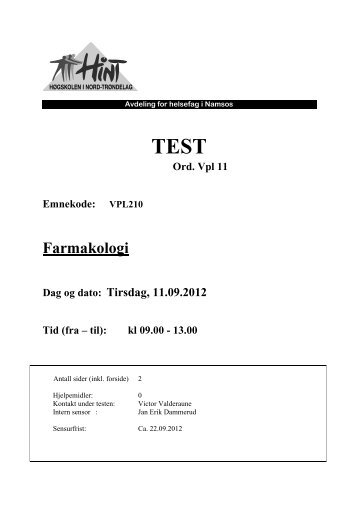The image appears to be a photocopy of an official document or form, predominantly in black and white with various shades of gray. It includes a logo of a company named Hint (H-I-N-T) positioned at the top left, featuring a triangle symbol which might depict skaters or dancers. Underneath the logo, there are several sections of black text, some of which read "ORD" and "VPL-11." The document, dated September 11, 2012, appears to be written in a language other than English, potentially German. The content of the text hints at an event confirmation related to a pharmacology test, detailing the date, time range, and additional reference numbers. The layout suggests it is formatted similar to a memo or letter, with clear and well-organized sections.